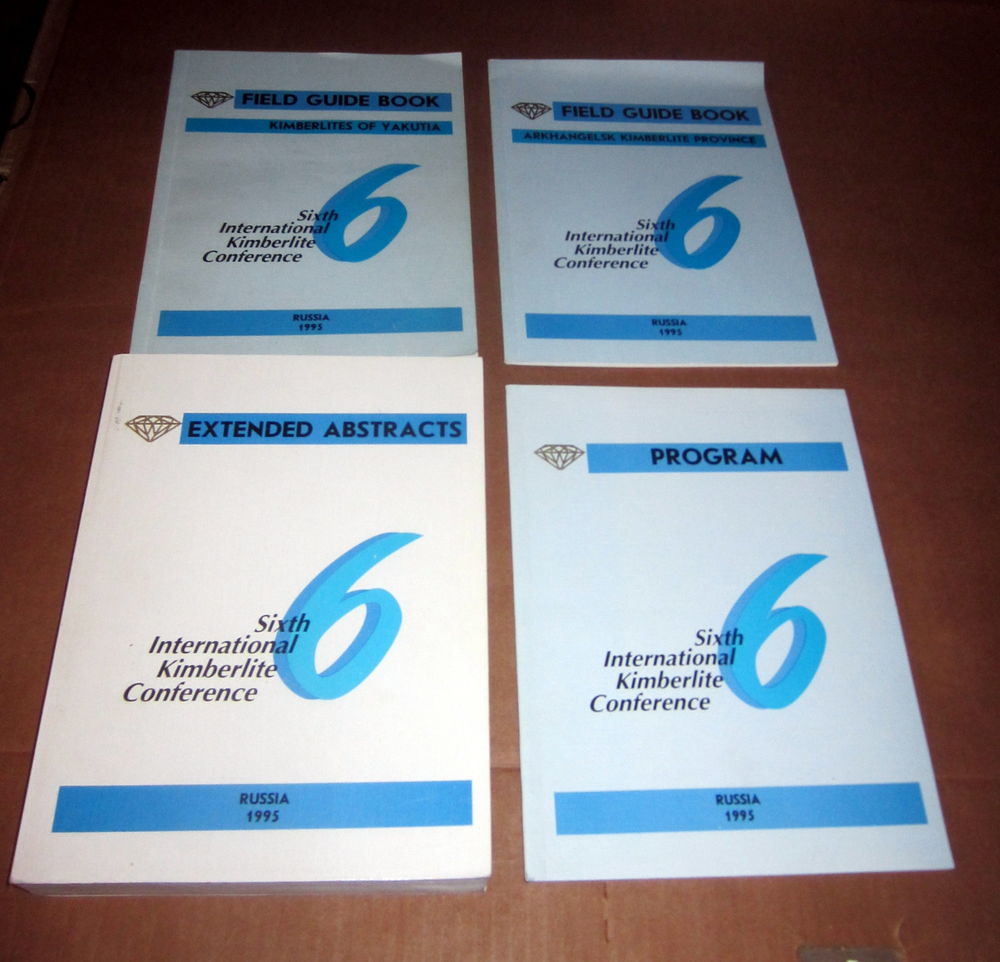The image depicts a photograph of four academic conference documents meticulously arranged on a brown wooden table, forming a square layout with two documents on top and two on the bottom. Each document features a consistent cover design: a large, blue-shaded number "6" positioned centrally, denoting the "6th International Kimberlite Conference." Above the number, there's a simplistic drawing of a diamond in brown at the top corners, and below the number, a blue bar spans nearly the full width of the documents with the words "Russia 1995" inscribed in black. The documents are titled differently—two titled "Field Guide Book" occupy the top positions, while the bottom documents are titled "Program" and "Extended Abstracts" respectively. The photograph captures the objects at a slight angle, giving a sense of depth and perspective.